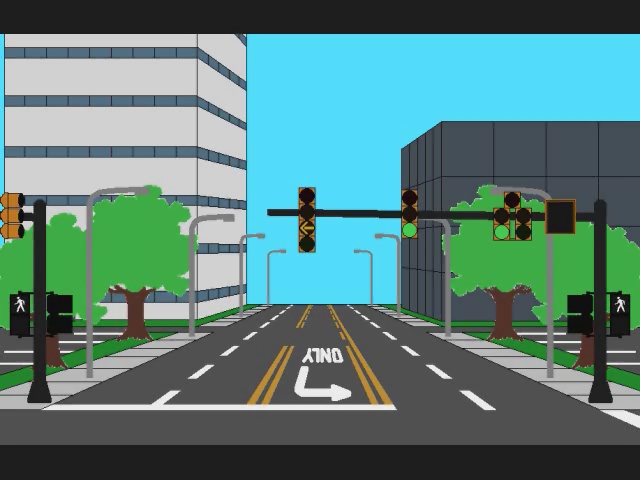This image is a computer-generated, simplistic animation of a city street intersection, resembling a scene from a video game. The focal point is a stoplight with three lights: a yellow arrow pointing left, and two green lights to the right. The light pole extends down to the sidewalk, which shows an illuminated white pedestrian signal indicating it's safe to walk. The gray sidewalk is neatly divided into perfect squares, with light posts spaced at regular intervals.

The road, depicted in gray, features a white dashed line running down its center, bordered by double yellow lines marking the turn lane directly underneath the yellow arrow stoplight. This turn lane has an arrow pointing left from the driver's perspective. There are additional white dashed lines as one moves left on the road, leading to another stoplight on a pole, reinforcing the intersection layout.

Surrounding the intersection, there are green trees on both sides, and two prominent buildings in the background: a large white skyscraper on the left and a shorter, four-story gray building on the right. The left side also features a parking lot in front of the skyscraper. The skyline is rendered in a solid turquoise-green color, creating a simplified backdrop. The image itself has a landscape orientation, cropped by black bars on the top and bottom.